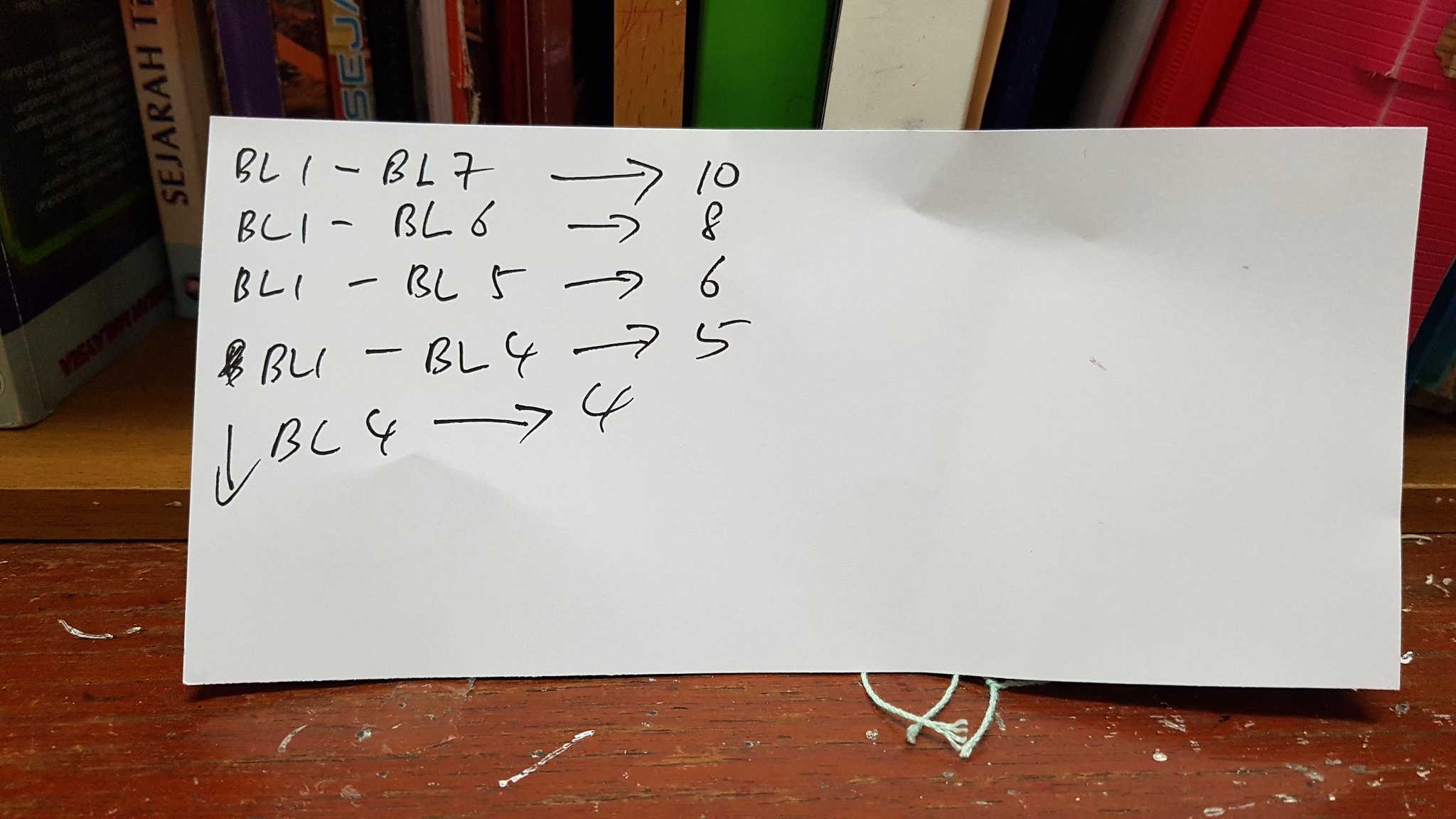A piece of paper, propped against a bookshelf, displays a series of handwritten instructions: 'BL1-BL7 Arrow 10, BL1-BL6 Arrow 8, BL1-BL5 Arrow 6, BL1-BL4 Arrow 5, BL1-BL4 Arrow 4.’ A small scribble is noticeable beside the final row. The wooden surface on which the paper rests is scratched and has a couple of thin white strings scattered beneath the document. The shelf behind the paper holds books of varying sizes; on the left, thin spines are visible, with one identifiable book named 'Sejarah' sporting a white cover. On the right, the larger spines suggest the presence of binders or similarly sized volumes.